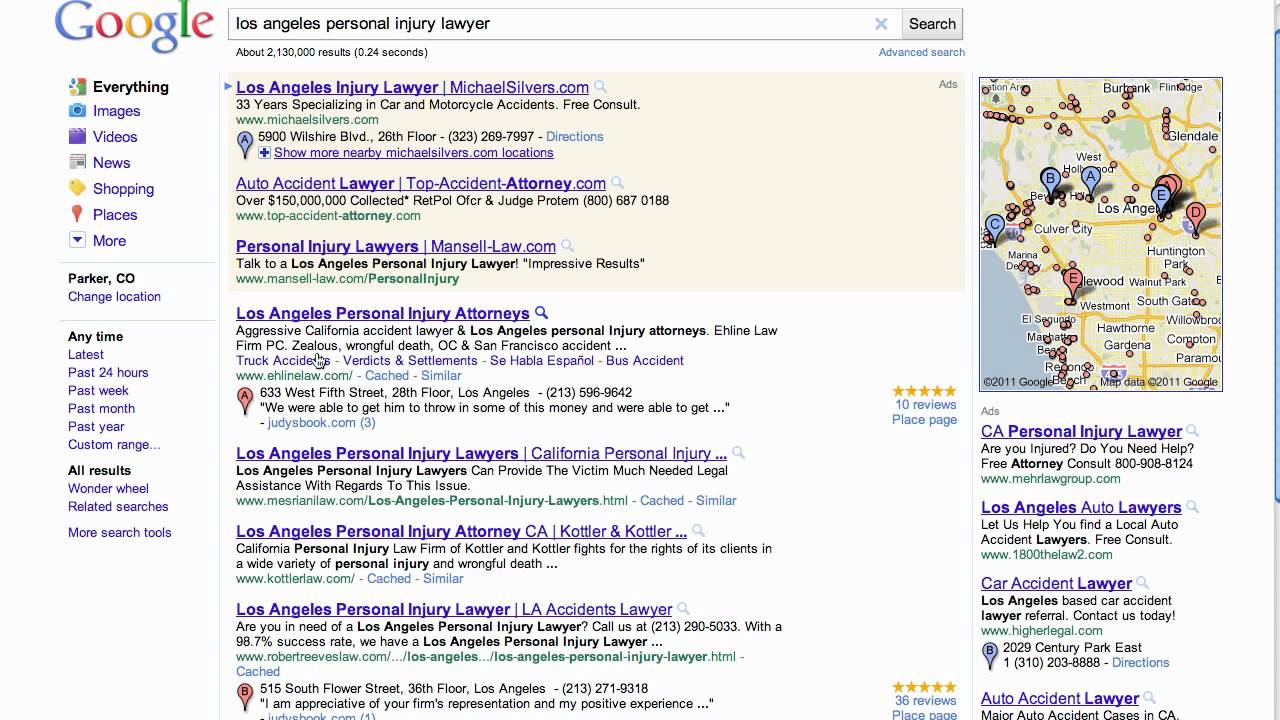Screenshot of a vintage Google search page interface: On the left side, the iconic Google logo is displayed prominently, alongside a menu bar with search category options: Everything, Images, Videos, News, Shopping, Places, and More. Below this menu, the location is set to Parker, Colorado, with an option to modify it. Time and results filtering options are presented further down.

In the center of the screen is the main search section, where the query "Los Angeles personal injury lawyer" has been entered. The search results display a mix of advertisements and organic listings, starting with a few sponsored ad results at the top. Below the ads, a series of listings for different Los Angeles personal injury lawyers are shown.

On the right side of the screen is a map highlighting the Los Angeles area, pinpointing the locations of the various law firms mentioned in the search results. Below the map are additional ads related to similar search phrases, such as "California personal injury lawyer."